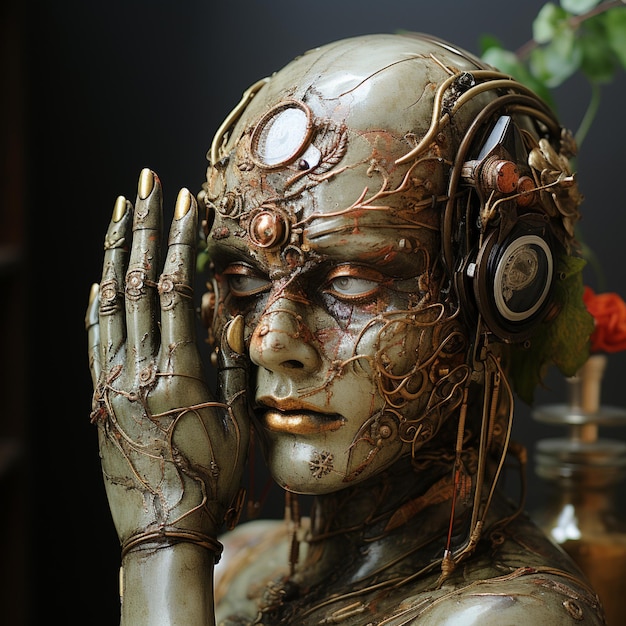This digital artwork showcases a detailed female humanoid robot with metallic, grayish-green skin adorned with vine-like copper wiring intricately embedded on her face, neck, shoulders, and hands. The character has pronounced, feminine features including gold eyelids, golden lips, and gold-polished nails. She is seen raising her left hand, partially covering the left side of her face, revealing more wires and ornate, jewel-like joints at her finger connections. Her bald head emphasizes a central feature on her forehead. The eyes are a captivating mix of gray and hazel. The background is predominantly dark and blurry, with a noticeable rose and some leaves on the right side, adding a touch of organic elements to the scene. This visually arresting image seems crafted for a film, capturing the essence of an alien or advanced AI being, blending human and futuristic robotic aesthetics expertly.